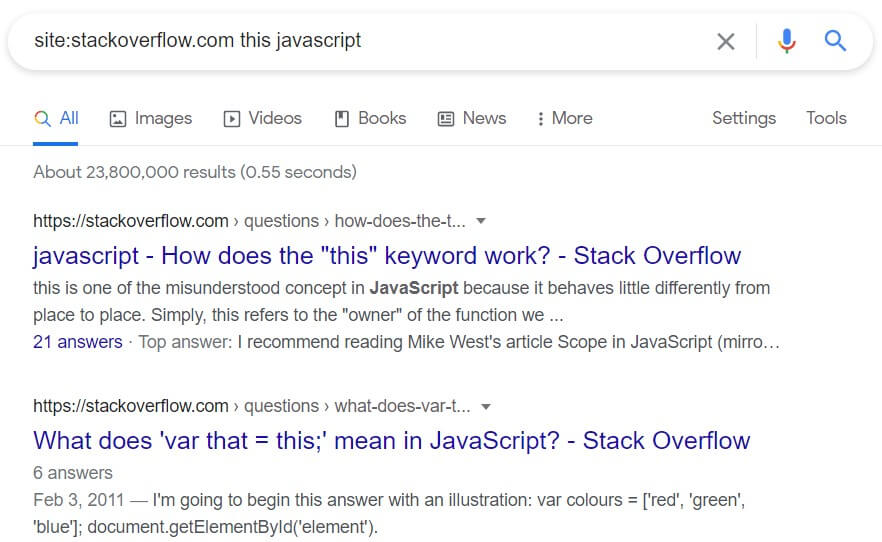This image captures a Google search results page. At the top, the familiar Google search bar is prominently displayed alongside the "Google Search" button. The search query appears to be related to JavaScript topics on StackOverflow.com. 

To the side of the main search area, there are several navigation tabs such as "All," "Images," "Videos," "Books," "News," and a "More" dropdown indicated by three dots.

Below the search bar, the results summary shows approximately 23,800 results, retrieved in 0.55 seconds (displayed in parentheses). 

The first two search results come from StackOverflow, appearing under a section dedicated to user questions. The first result addresses a question titled, "How does the 'this' keyword work in JavaScript?" The second result pertains to, "What does 'var that = this' mean in JavaScript?"

These concise yet informative search result entries align with typical searches for coding-related queries, providing quick access to relevant discussions and solutions from the StackOverflow community.